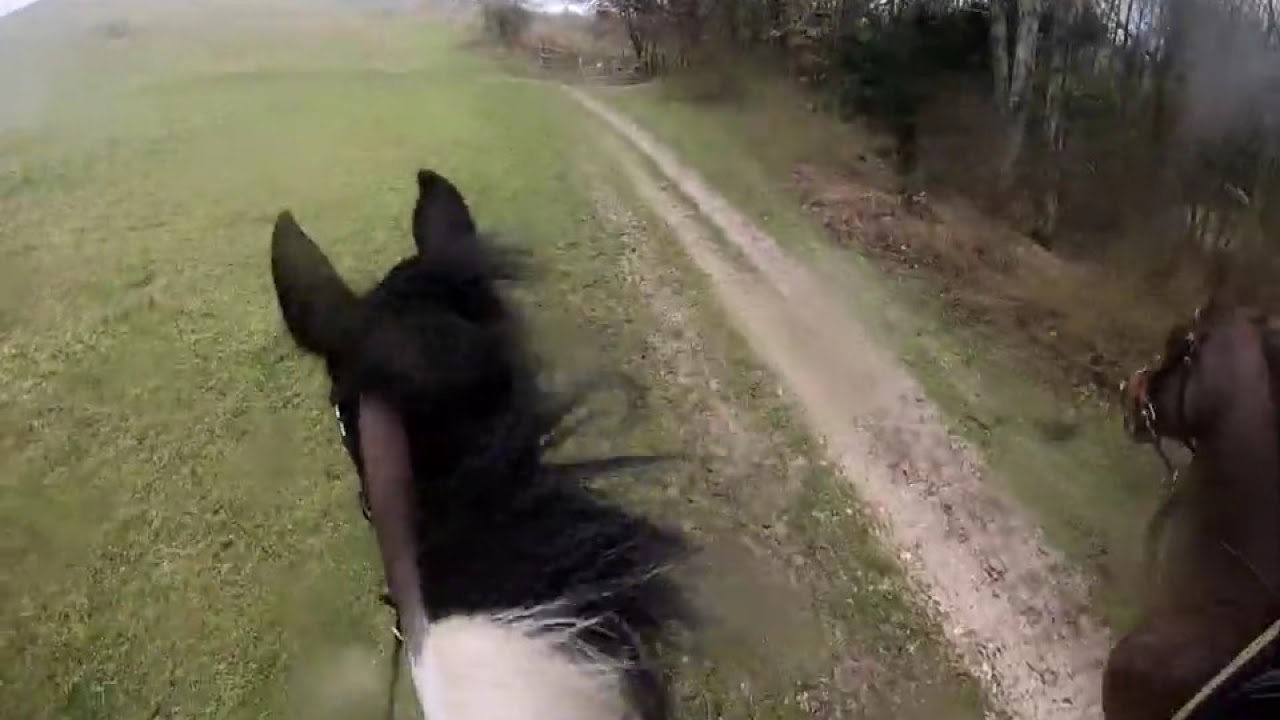In this horizontally aligned, rectangular image, we see a scene that is notably blurry, possibly due to water droplets or condensation on the lens, suggesting a rainy or misty day. The foreground is dominated by two horses, viewed primarily from behind. On the left, the horse has striking black pointy ears, a black mane with some white near the base, and a brown coat. The right horse has a brown coat and is equipped with a saddle, but its mane is not visible. Both horses appear to be positioned as though pulling a carriage or someone down a gravel path that runs diagonally upward from the bottom right towards the top center of the image. Flanking this path is a stretch of green grass, with more grass evident on the left side of the frame. The right side features a corner of dense woods characterized by tall, slender, leafless trees, potentially birch. In the background, a rustic fence lines the gravel path, leading towards the indistinct, whitish sky. The overall atmosphere of the picture evokes a calm, albeit dreary day, with the landscape shrouded in a gentle haze accentuated by the blurred focus of the photograph.